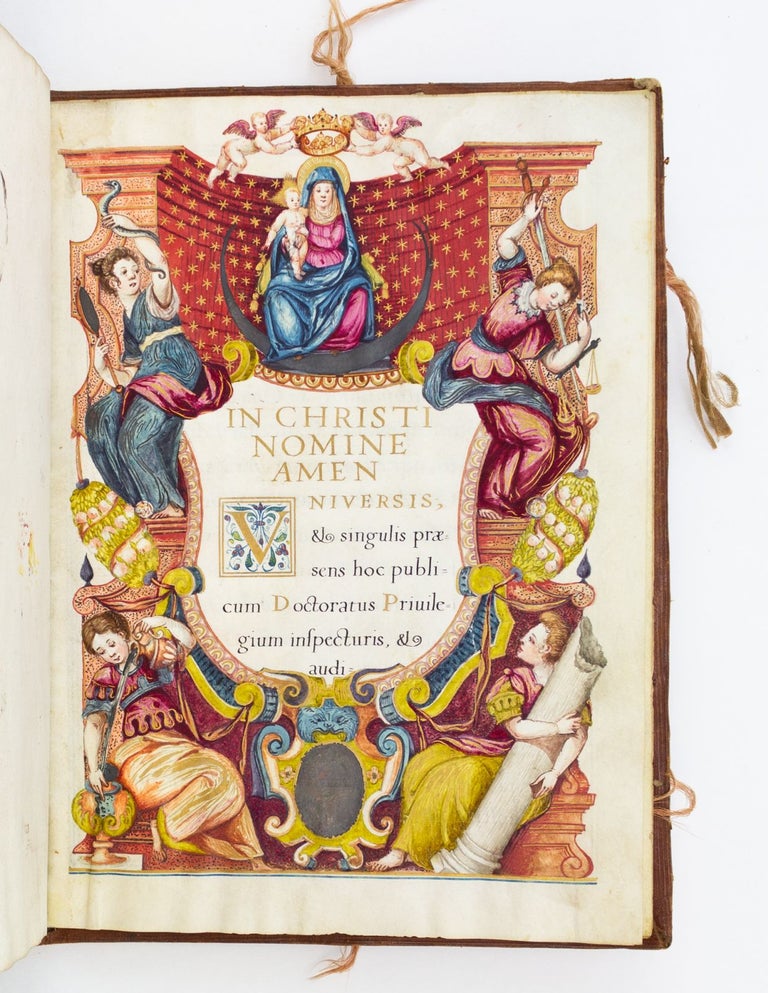The image is of an old, wrinkled and stained page from a Latin Christian text, possibly from the Bible, mounted on a brownish background with a few strings hanging from the right side and bottom. The illustrated scene features the Virgin Mary in a purple dress with a blue cover, sitting with Baby Jesus in her arms, and a crown above her head held by cherubs or angels. Surrounding them are four women, two on each side: the woman on the upper left holds a mirror, while the upper right woman holds a downward-pointing sword and scales. Below them, the lower left woman appears to be pouring liquid into a container, and the lower right woman grips a broken column. The center of the page contains a shield-like shape with the Latin text "In Christi Nomine Amen Universis," indicating the religious nature of the document. Red accents and stars are visible behind Baby Jesus and the Virgin Mary, adding to the detailed and intricate artwork.